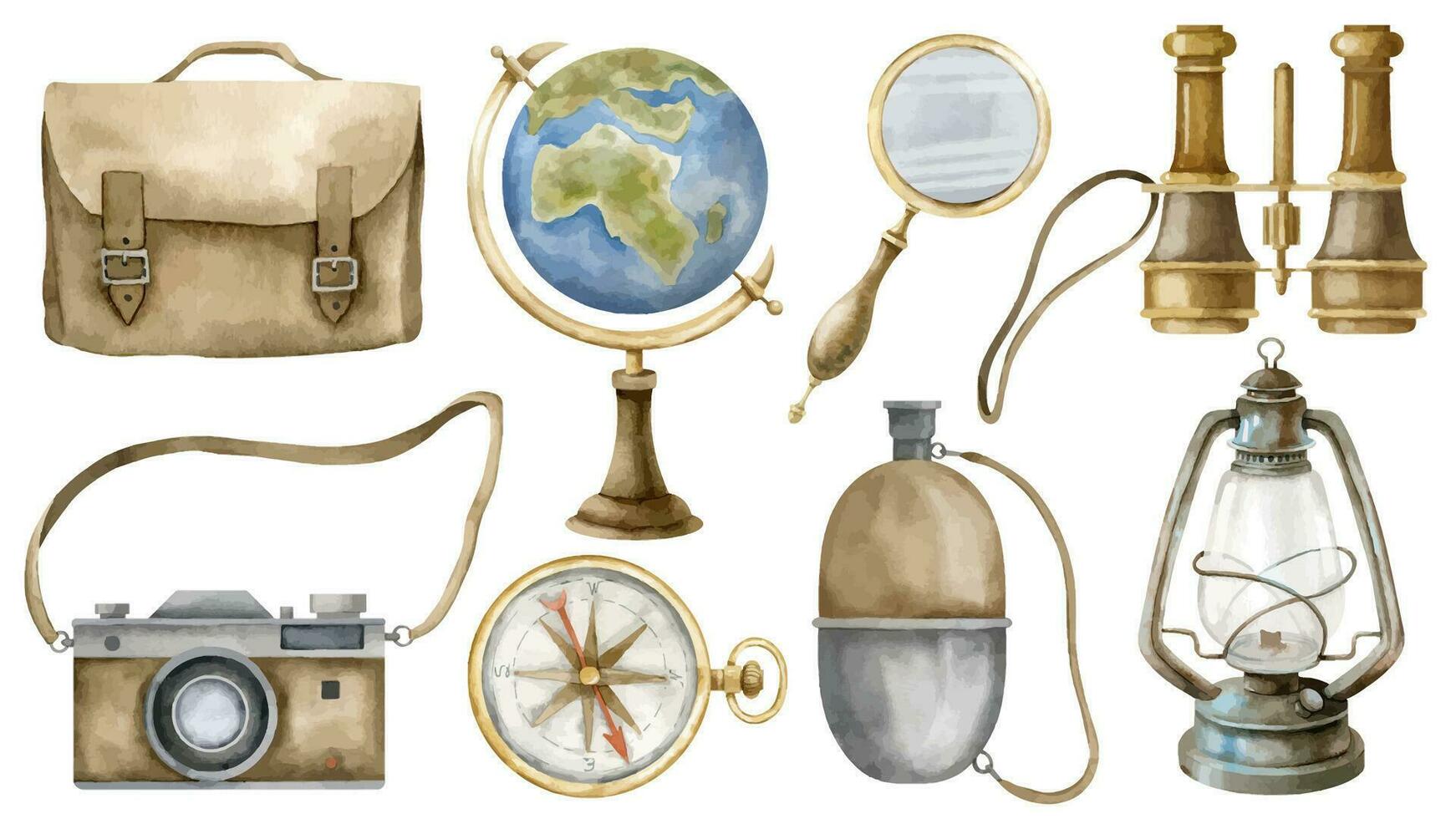This detailed illustration, featuring a hand-painted watercolor finish in neutral tones, depicts a collection of vintage travel items meticulously arranged in two evenly spaced rows. In the top left, there's a tan briefcase with brown handles and silver buckles, reminiscent of something you'd use for papers or folders. Adjacent to it, to the right, is a globe held by a gold crescent base descending into a wooden stand, merging into the same beige tones. Alongside the globe, further right, is a diagonally positioned magnifying glass with a wooden handle and gold trim. At the far right of this row, a pair of old-fashioned binoculars, seen from the top, completes the top row. Below, starting from the left, there's a vintage film camera with a conspicuous brown strap, facing directly at us. Next to the camera is a gold-trimmed compass featuring red and brown direction indicators. Following it is a beige and silver canteen with a gray stopper, and lastly, a silver and glass oil lamp sits directly below the binoculars, mirroring the aesthetic of a seasoned explorer's toolkit.